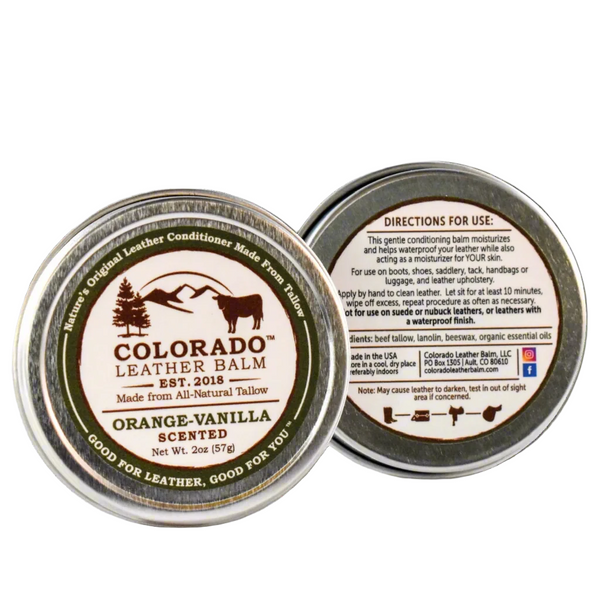The image features two cylindrical metal tins with a chrome finish, set against a plain white background. The tin on the left displays the front label in full detail, while the tin on the right is partially obscured, revealing the back label.

The front label of the tin on the left exhibits a detailed design. At the top, "Colorado Leather Balm" is printed in bold brown text, followed by "EST 2018" on a brown line. Directly beneath, the text states "made from all-natural tallow." There is a dividing brown line, below which "Orange Vanilla" is written in dark green, followed by "scented" in brown. The net weight is listed as "2 oz (57 grams)" in brown text. Surrounding this text is a tan-colored outer ring which reads "Nature's Original Leather Conditioner made from tallow" at the top and "Good for Leather, Good for You" at the bottom. The center of the label features a brown illustration of mountains with sunbeams emerging from behind, flanked by conifer trees on the left and a cow on the right.

The back label, only partially visible on the right tin, contains detailed usage instructions and additional information in brown and black print. It starts with "Directions for Use" in brown, followed by instructions in black: "This gentle conditioning balm moisturizes and helps waterproof your leather while also acting as a moisturizer for your skin. For use on boots, shoes, saddlery, tack, handbags, or luggage, and leather upholstery, apply by hand to clean leather. Let sit for at least 10 minutes. Wipe off excess. Repeat procedure as often as necessary." A cautionary note in dark black reads, "Not for Use on Suede or Nubuck Leathers or Leathers with a Waterproof Finish." Ingredients listed include beef tallow, lanolin, beeswax, and organic essential oils. Additional text states it is made in the USA and advises storing in a cool, dry place. The label also provides the company’s address: "Colorado Leather Balm, LLC, PO Box 1305, Alt, Colorado, 80610," and the website "coloradoleatherbalm.com." A final note in brown warns: "May cause leather to darken. Test in out-of-sight area if concerned."

Both tins convey a meticulous attention to detail, emphasizing the product’s natural composition and effectiveness in leather care.